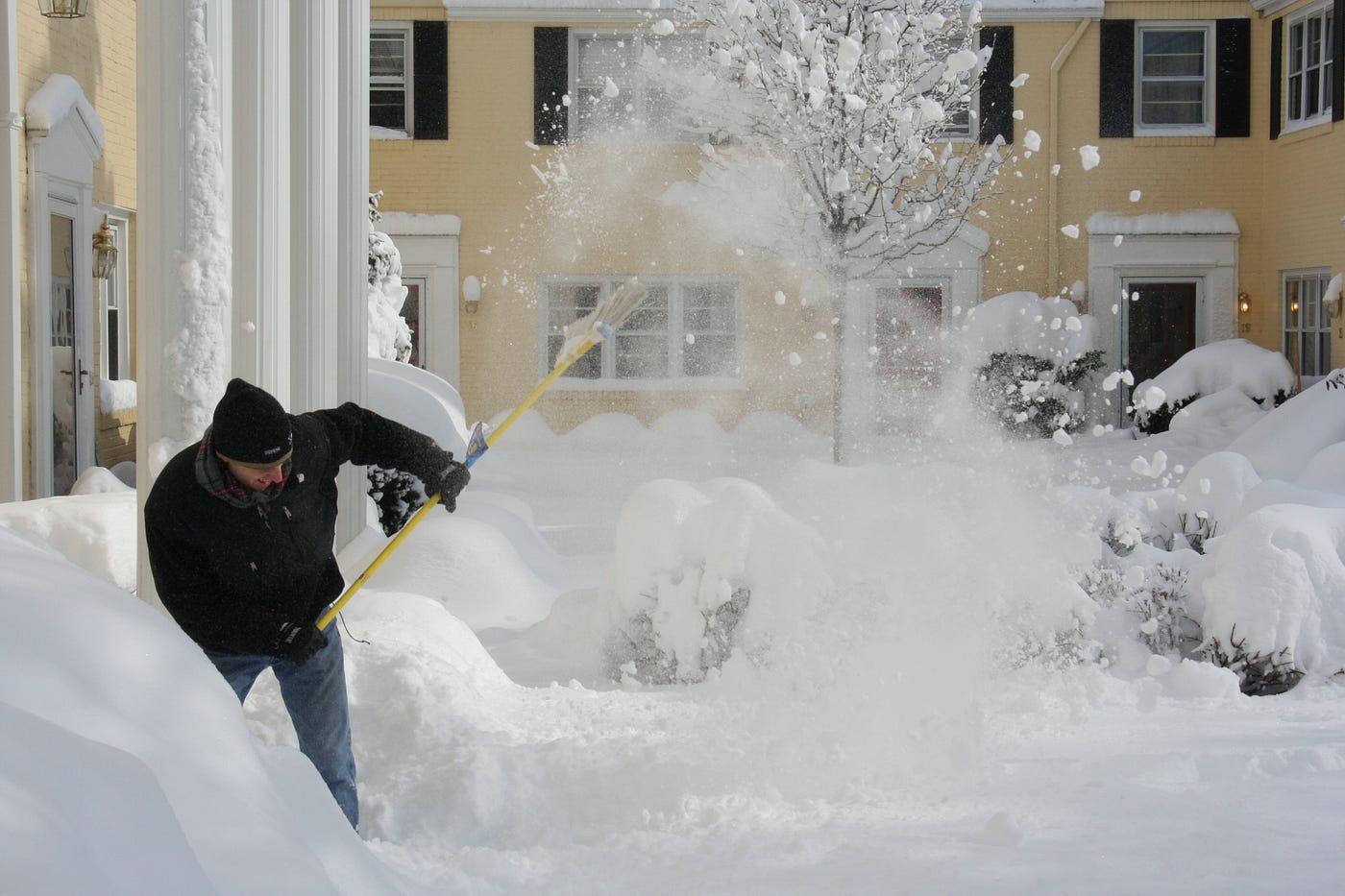The photograph captures a man tirelessly working to clear snow from his knee-high, snow-covered porch using a yellow-handled broom amidst a winter setting that suggests the aftermath of a blizzard. He is caught in mid-motion, sweeping the powdery snow into the air. The man is dressed warmly in a black knit cap, a black jacket or coat, blue jeans, and gloves, possibly wearing a small scarf or benefiting from his jacket’s collar.

Behind him stands an ornate, yellow-colored building with white trims, which could be an apartment complex. The structure is detailed with multiple entry doors adorned with elaborate moldings and flat windows, some featuring black shutters. Prominent white columns frame the area where he is working, and small lights embellish the sides of the doors—one glowing softly with an orange hue. Bushes, nearly buried under the thick snow, sporadically punctuate the courtyard, while a tall tree in the background is heavily laden with snow, all illuminated by the sunlight of a clear day.